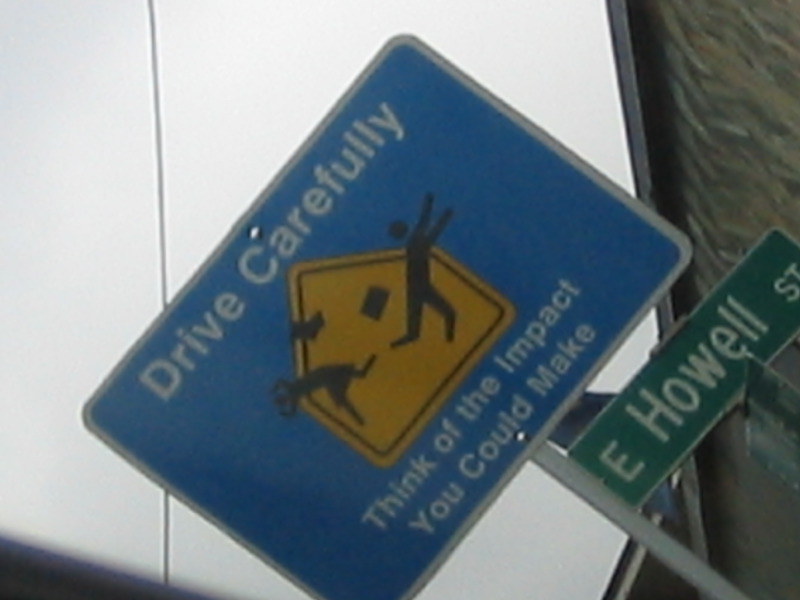The image captures an exterior scene at a sharp angle, focusing on a street sign. The background is predominantly a hazy, light gray, contributing to an atmosphere of indistinctness. Emerging from the lower right corner and extending upwards towards the left, the pole immediately draws attention. At the top of the pole sits a prominent blue sign with a white border. Centrally, this blue sign features a yellow, house-shaped warning icon bordered in black, depicting two figures seemingly in mid-air collision — one flying rightwards, the other leftwards, as if they have been struck. Above this cautionary image, white text commands, "Drive Carefully," while below it reads, "You Can Make." Further down, attached to the right side of the pole, a green rectangular sign clearly labels the street as "East Howell Street."